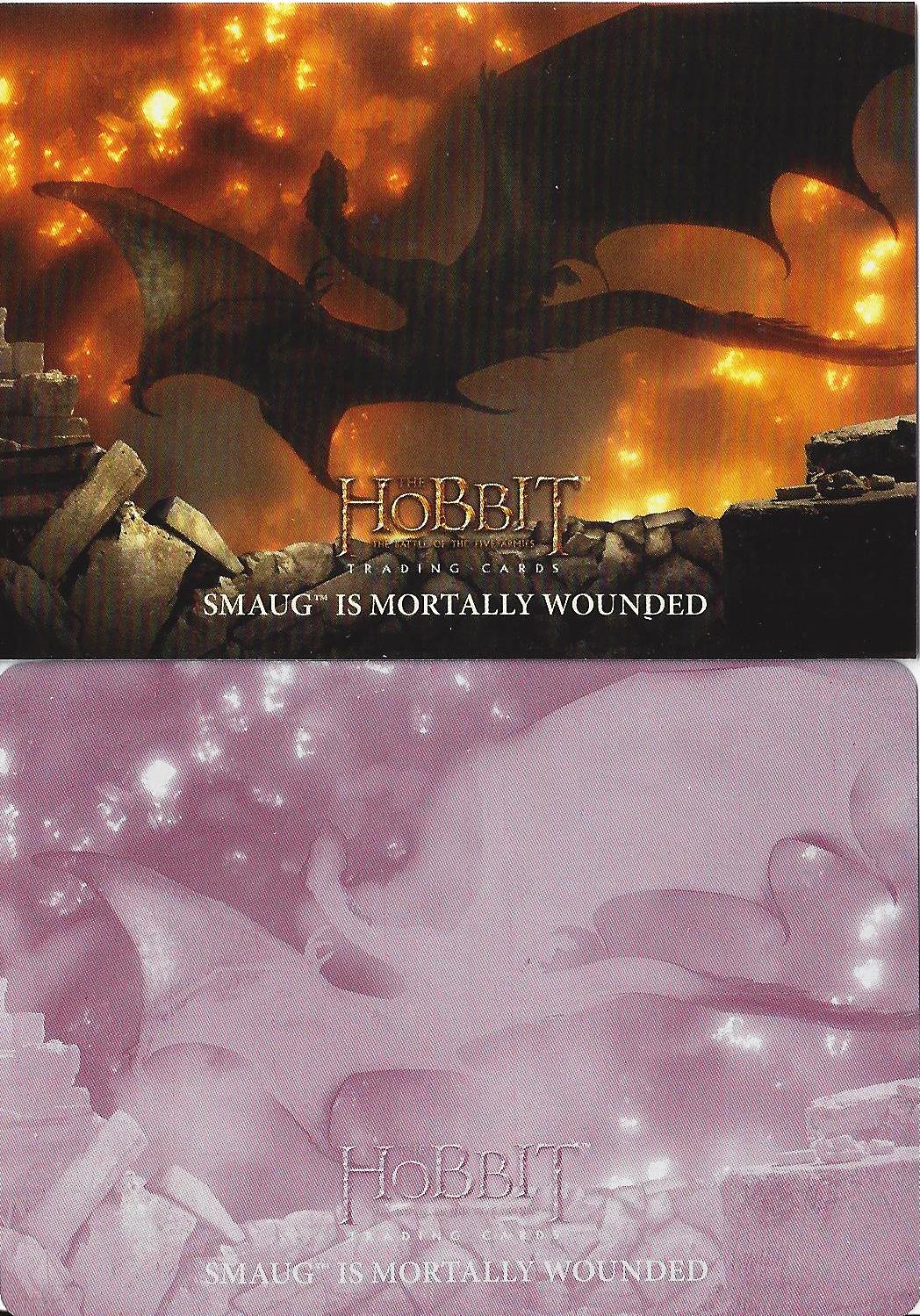The image depicts a scene from "The Hobbit," specifically showing the dragon Smaug mortally wounded. The picture appears twice, one above the other, each with distinct visual treatments. The top image is a detailed and colored still, featuring a partially illuminated dragon, with Smaug appearing brown against a backdrop of burning fires and swirling smoke. Rocky terrain can be seen in the foreground. The text on the image reads: "The Hobbit," followed by "Trading Cards," and below that "Smaug is Mortally Wounded." The bottom version of the same image has a negative effect, with the entire scene rendered predominantly in pink and red hues. This altered version still bears the same descriptive text, but the colors suggest an evolution from its initial, perhaps unfinished state.